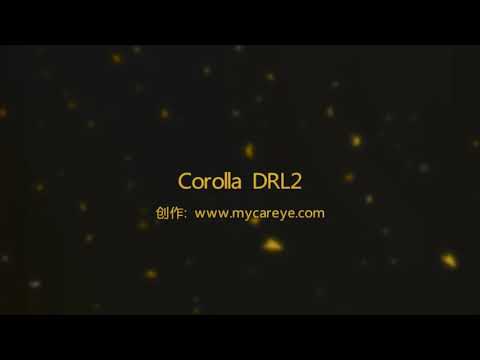The image appears to be an edited or animated graphic featuring a plain black background adorned with sporadic, bright gold flakes scattered throughout. At the top and bottom of the image, there are black bars each occupying about an eighth of the page. Centrally located on this textured backdrop, the word "Corolla" is displayed in all lowercase, followed by "DRL2" in capital letters. Beneath this primary text, in a smaller but matching gold font, there are Chinese or Japanese characters, followed by the website URL "www.mycareye.com." The gold lettering stands out distinctly against the dark, star-like background, emphasizing the main visual elements amidst the subtly illuminated specks. This image likely originates from a website or digital source and contains no other objects or people.